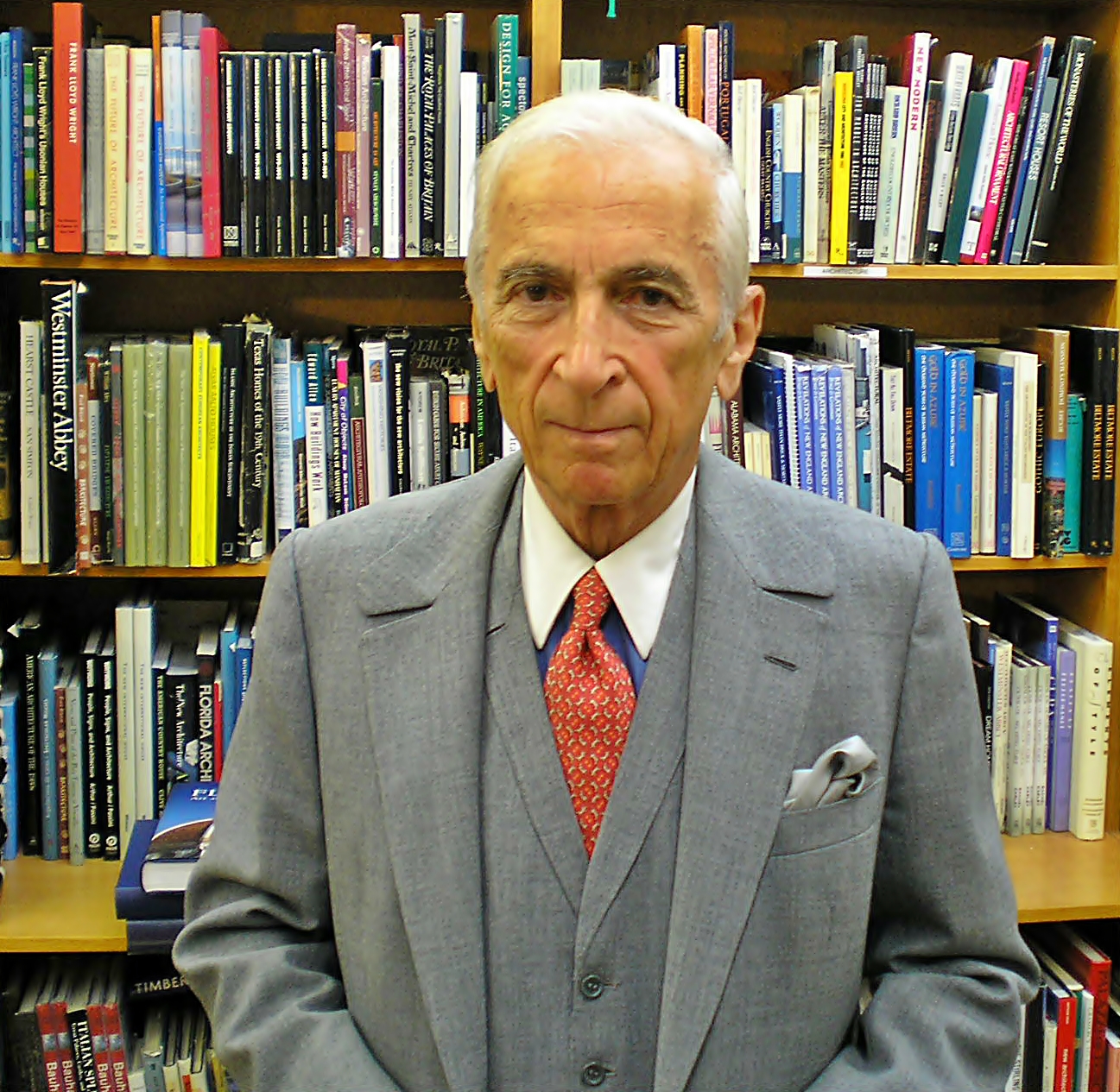The photograph features an elderly white man, likely in his late 60s or 70s, standing directly in the center of the image. He is dressed in a sophisticated, gray suit paired with a matching gray vest. His blue shirt, notable for its thick white collar, complements his red tie adorned with white and orange specks. The man has white hair, parted to the left and combed over to the right, with thinning at the front. His bushy, wiry grey eyebrows frame his clean-shaven, heavily wrinkled face, which bears a subtle smile. He looks directly at the camera, creating a focal point amidst the richly detailed background. Behind him, a four-tiered bookshelf brimming with meticulously arranged books dominates the scene. Titles like "Westminster Abbey" and something related to Florida are discernible among the countless colorful spines, ranging in hues of blue, orange, red, dark blue, white, tan, light green, brown, and black. The setting appears to be a library, captured indoors in the middle of the day, offering a scholarly and nostalgic atmosphere.